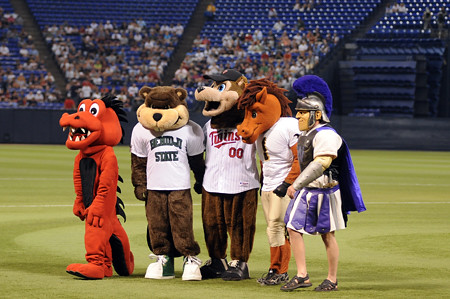This vibrant photograph captures a lively gathering of mascots at a sporting event in a stadium. The scene is set on green turf, with large blue bleachers in the background, half-filled with spectators. Visible in the bleachers are slanted aisles leading upwards. The mascots are lined up for the photograph, representing various teams. From left to right, there's an orange alligator mascot facing left, a bear wearing a white shirt reading "Bemidji State," and another character, possibly a wolf, donning a white shirt with the word "Twins" in red. Next is a horse mascot looking to the left, clad in a white shirt. The lineup concludes with a striking Roman gladiator or Spartan figure, adorned in a silver helmet with a blue plume, complemented by a blue cape and belt. The collective presence of these diverse mascots, ranging from a tiger to a Trojan man in full armor, emphasizes a rich blend of team spirit amidst a bustling sports event.